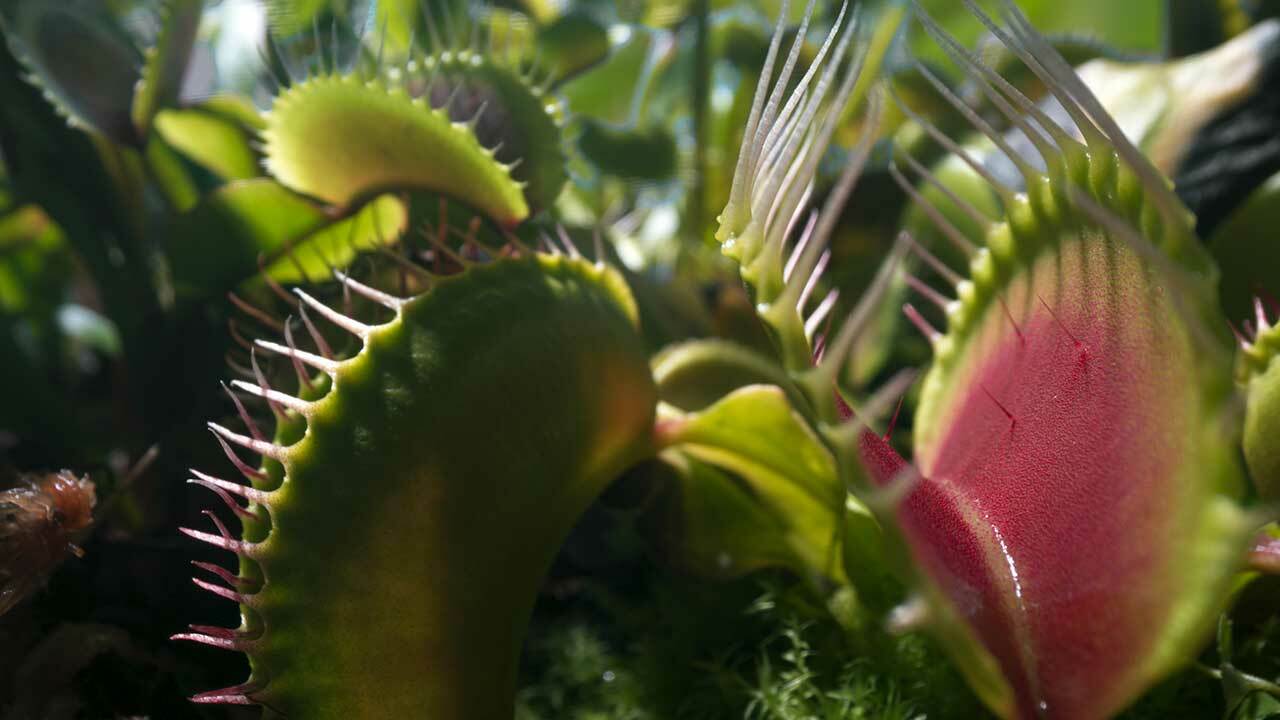This detailed close-up image captures the fascinating intricacies of a Venus flytrap in a lush, green, jungle-like environment during a bright, clear day. Prominently featured on the right side of the frame is an open Venus flytrap, its vibrant green outer edges contrasting starkly with the striking fuchsia-pink and beige hues inside its “mouth.” The edges of the plant are lined with long, white spikes that curve inward at about a 45-degree angle, resembling tentacles or teeth, prepared to ensnare unsuspecting prey. On the left side, another Venus flytrap is closed tightly, its interlocked spikes forming a cage-like barrier, possibly containing an insect. The background, although slightly out of focus, reveals more Venus flytraps and foliage, enhancing the jungle-like atmosphere of this remarkable macro perspective, vividly showcasing the plant's unique hunting mechanism.